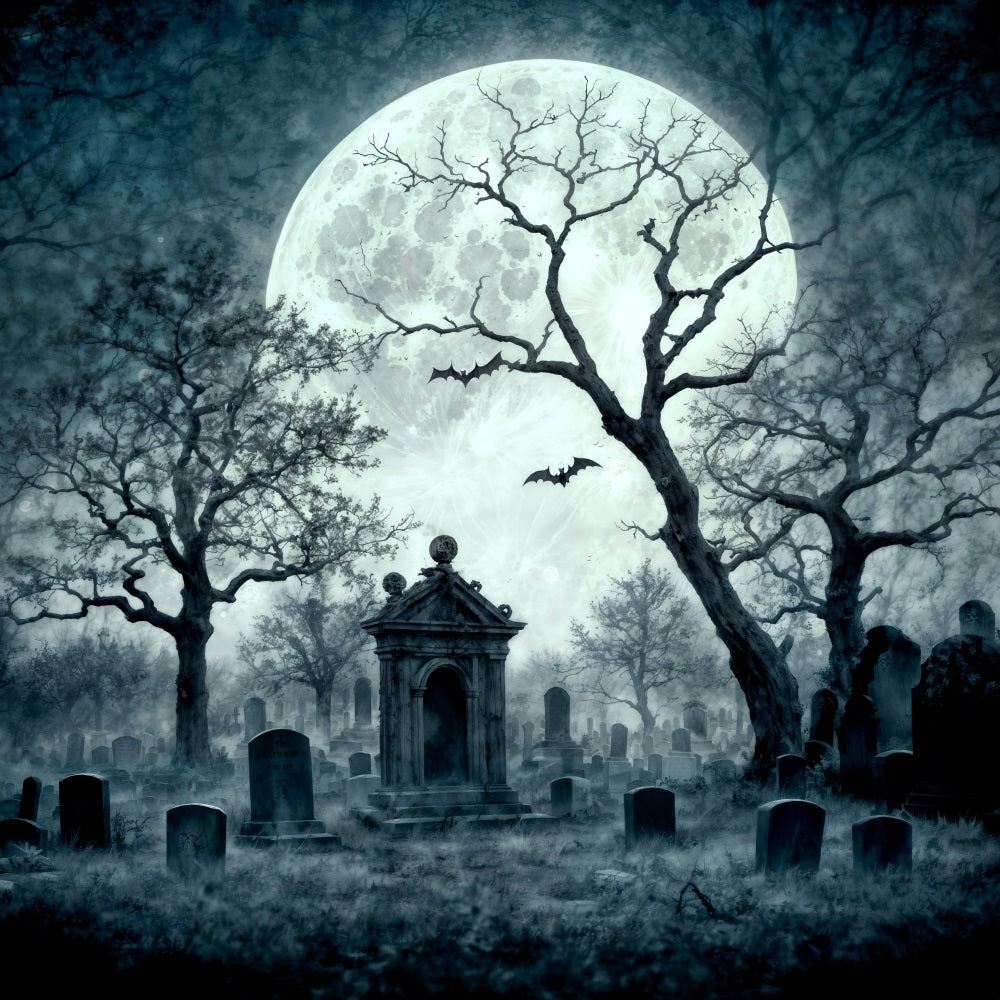This eerie, black-and-white illustration captures a haunting Halloween scene set in a graveyard under a radiant, full moon. The centerpiece of the graveyard is a large, prominent headstone that resembles a doorway with a triangular top, surrounded by numerous smaller headstones scattered throughout. The moon, which dominates the background, showcases detailed spots and craters, and its glowing light bathes the entire scene in a chilling luminosity. Silhouetted against the bright moon are two bats in flight, adding to the spooky atmosphere. Three leafless, withered trees stand tall in the foreground, with additional tree silhouettes fading into the background, enhancing the scene's depth and desolation. The image also features patches of grass and scattered twigs on the ground, and the corners darken towards the edges, creating a vignette effect that heightens the overall ominous feel.